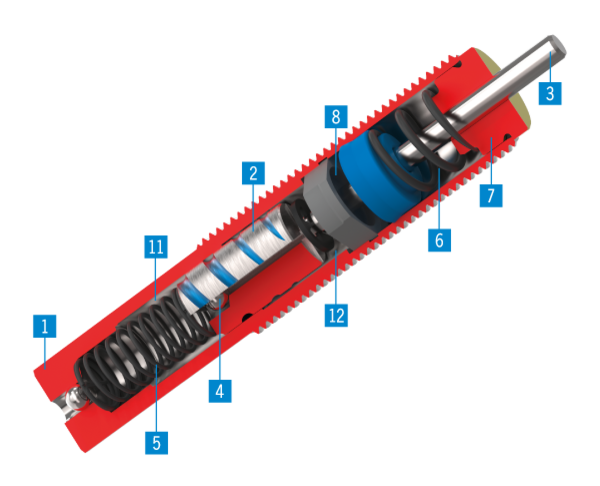This image depicts a key component for a specific apparatus. The uppermost section of the component is orange, and directly beneath it, a metal rod is securely attached. This metal rod runs through several other pieces. Among these pieces is a blue circular element, followed by another round piece that is a dark charcoal black color, resembling wheels. At the far end of the setup, there is a substantial black spring, essential for the device's functionality. Surrounding the device, numerical labels (such as 1, 2, etc.) are present, indicating and identifying the various parts of the mechanism for clarity and reference.